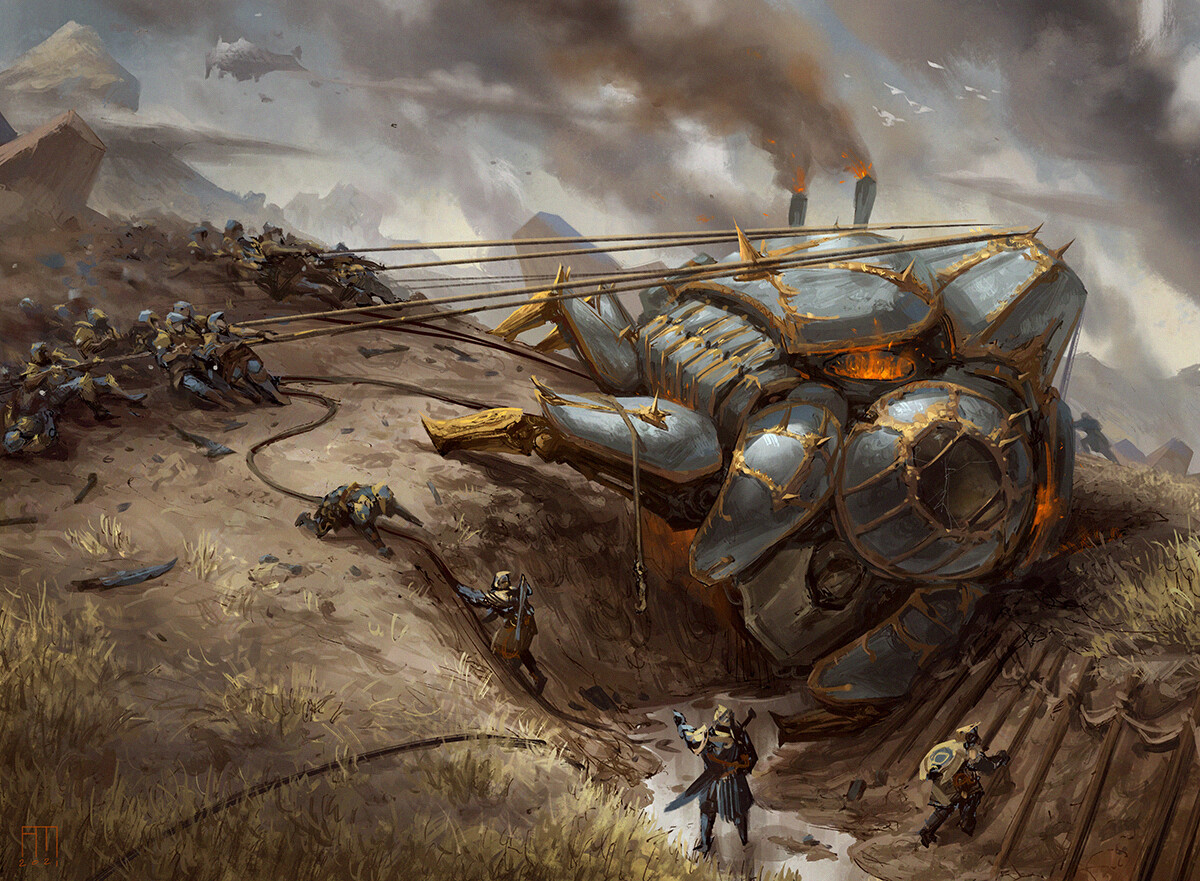The image depicts a detailed artwork of a futuristic scene set in an outdoor environment, dominated by a vast expanse of scattered dirt with traces of green grass. Central to the scene is a large blue spacecraft-like machine that appears to have crashed into a water-filled valley. The craft, which features a large round window, numerous panels with gold trim, and rectangular shapes, is being pulled upright by groups of soldiers in blue and yellow uniforms, distinguished by blue helmets and gold-trimmed gear. The soldiers utilize brown ropes to tug at the craft, which shows signs of internal fire with red flames visible through the panels. Background elements include a partially cloudy sky, distant smoke, and a snowy mountain peak. Additional figures in the background, adorned in robes and wielding swords, alongside others in the upper land level handling ropes, contribute to the bustling, chaotic atmosphere. The scene blends elements of battle and recovery, underscored by the machinery, human effort, and ominous environmental details.